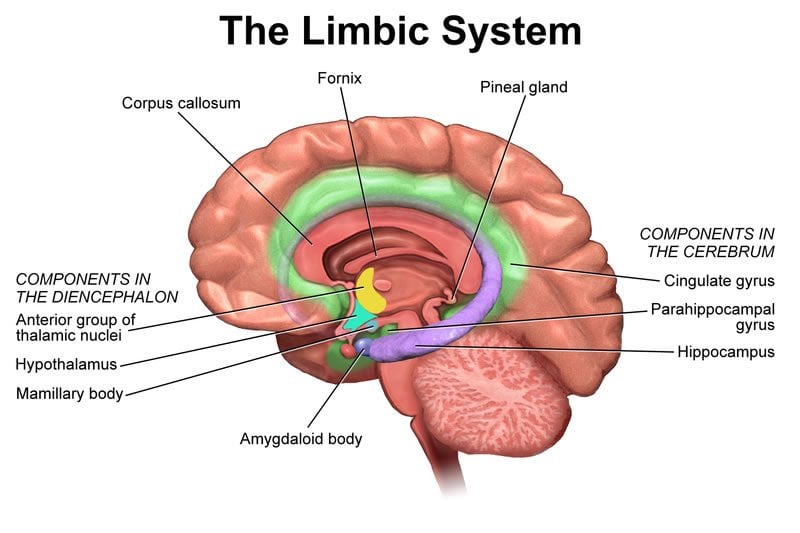The image displays a detailed, three-dimensional illustration of a brain cross-section set against a white background. Central in the image, a pink-colored brain showcases multiple layers, including a green layer inside the outer pink portion and a smaller purple layer within. Additionally, there are folded pink regions and a small yellow layer. The image is extensively labeled with black text identifying various parts of the brain, with lines pointing to each respective region. Prominently, the central text identifies the "Limbic System." Surrounding labels include "corpus callosum," "fornix," "pineal gland," "components in the cerebrum," "cingulate gyrus," "parahippocampal gyrus," "hippocampus," "amygdaloid body," "mammillary body," "hypothalamus," "anterior group of thalamic nuclei," and "components in the diencephalon." This image, part of a stylus medical imagery series, provides a comprehensive diagrammatic representation of the limbic system and its associated structures.